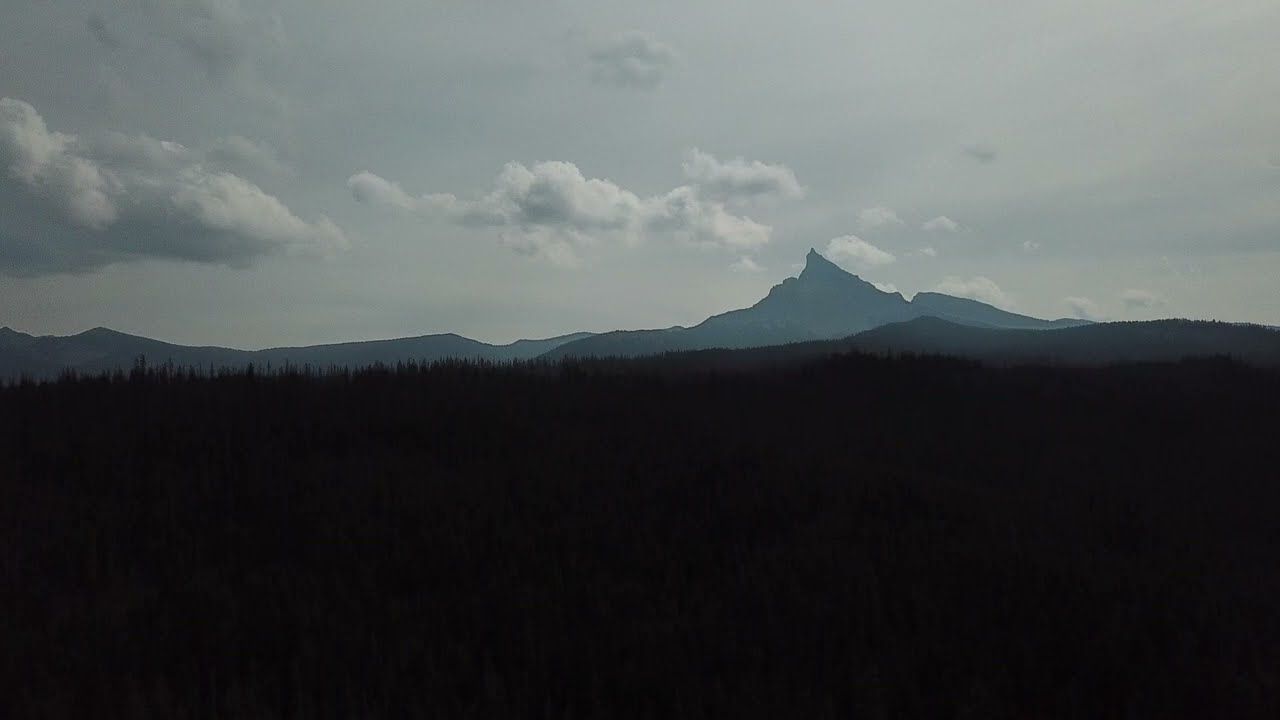The photograph captures an outdoor landscape at dusk, characterized by its overall dark and somber tones. The bottom half of the image is dominated by a silhouette of a forested, hilly terrain, shrouded in deep shadow and indistinct details. Rising towards the center of the image are rugged mountain peaks, their sharp, meringue-like tops silhouetted against the sky in a dusty, darkish blue hue. The sky above is a brooding, dark gray scattered with sparse, fluffy clouds, predominantly visible towards the middle and left of the image. The entire scene exudes a dreary and melancholy atmosphere, with the grayscale-like color palette accentuating the sense of dusk or possible image manipulation.